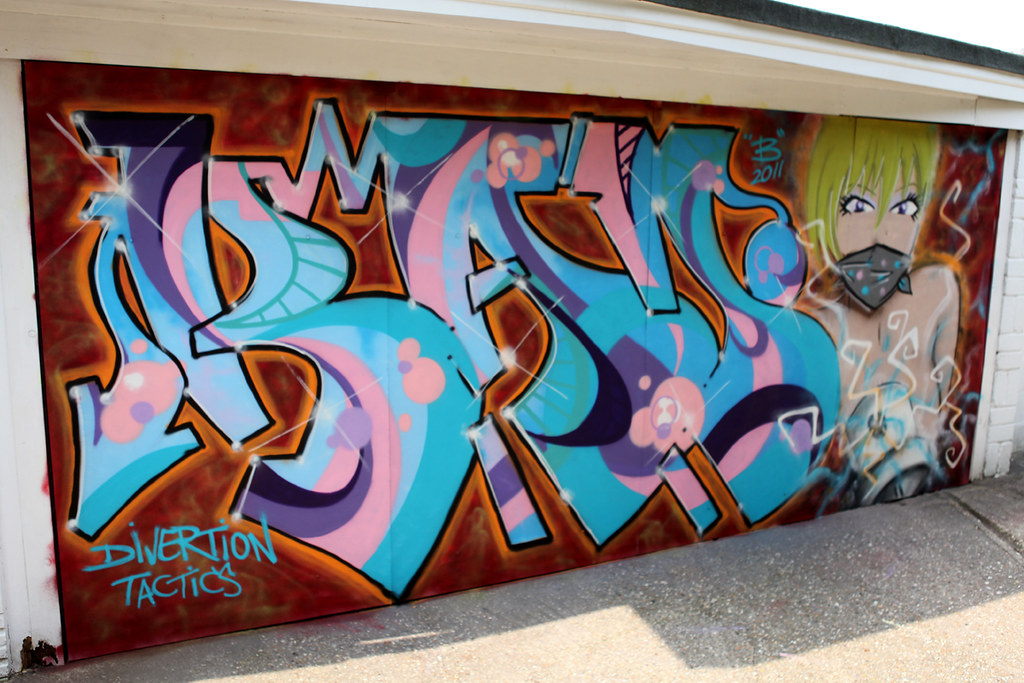The photograph captures the side of a white building, where a red garage door serves as the canvas for an elaborate piece of street art. The graffiti features a mix of swirling, unreadable text in vibrant hues of pink, purple, blue, teal, black, and light blue, highlighted with an orange glow. Dominating the right side of the door is a spray-painted image of a woman with short blonde hair, her face partially obscured by a dark gray bandana with blue and pink polka dots. She appears topless, holding a spray paint can from which squiggly lines are emanating. The graffiti is signed in light blue with the words "Diversion Tactics" at the bottom left, and above the woman’s head, it reads "BE 2011" in a subtle, intricate design.